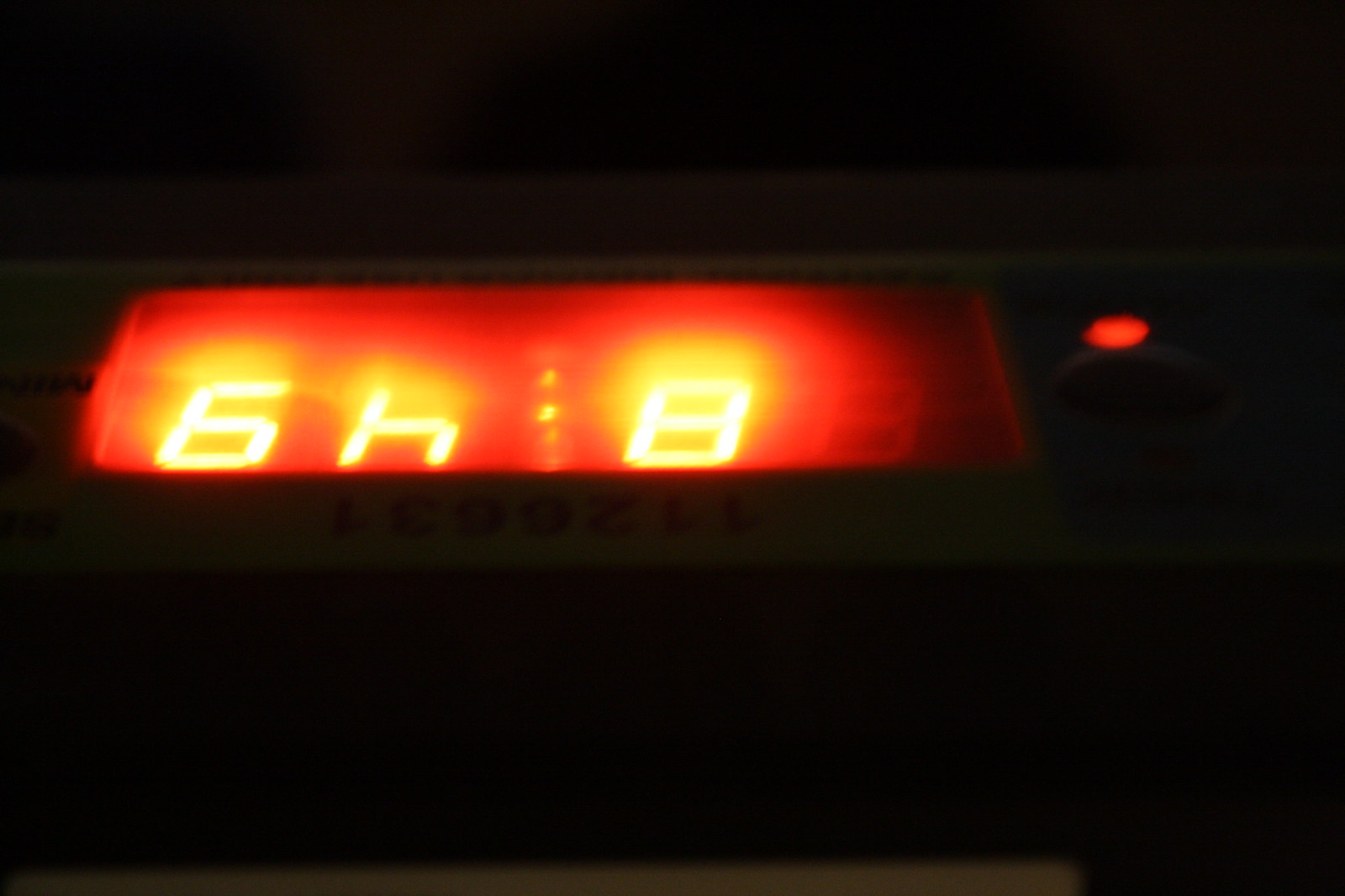In the darkness of a room, a lone digital alarm clock illuminates the surrounding area with its faint glow. The time displayed is "8:49" in red, though the clock appears to be upside down. A red button or indicator light is visible on the right side, adding another point of brightness. The clock's screen is framed by a white border, and it features some indistinct text, possibly the brand name, at the top. The red digits cast a subtle yellow halo around them, blending into the surrounding darkness, reinforcing the notion that it could be 8:49 PM in the depth of a winter evening.